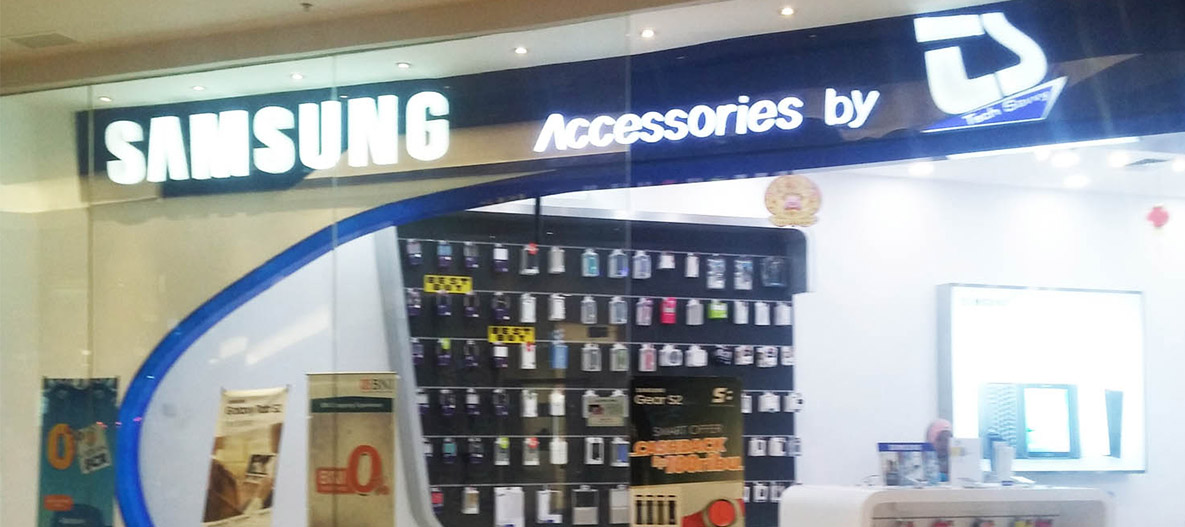This image depicts a storefront with a prominently featured white-lit sign on a blue background that reads "Samsung Accessories Buy," accompanied by a logo to its side. The storefront, potentially situated in a mall as suggested by the visible beige ceiling in the top left corner, reveals a glimpse of the interior through clear glass windows. Inside, the store is brimming with an array of phone accessories, displayed meticulously across several black display boards adorned with numerous rows of items, likely phone cases. Positioned centrally, a table holds various flyers or products, standing in front of a lit screen that predominantly displays a white advertisement, possibly for a tablet. The visibility of interior details is hampered by glare and blurriness, making finer elements challenging to discern. Distinct posters are affixed to the glass windows and walls, adding to the store's promotional atmosphere.